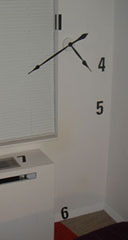The image depicts a small, seemingly unrealistic room. The room features a window with its blinds drawn down and a brown floor. A heater is positioned below the window. In the lower right corner, there is an indistinct black object. A unique element in the scene is the superimposed clock with long, pointed hands. The clock numbers are irregularly placed: the numbers 4 and 5 are positioned where they normally would be, but the number 6 is situated low on the floor, and the number 7 appears on the heater. The clock lacks numbers beyond these, with the only other marking being two lines at the position where the number 11 would typically be. The clock numbers and markings are all in black.